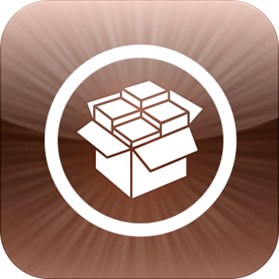The image appears to be an icon for a smartphone or tablet app. It is a round-cornered square with a background that transitions from a darker brown in the center to a lighter rose gold hue at the top and bottom, giving the effect of radiating rays. The icon has a thin white circle in the middle, which emanates faint white "fingers" extending outward slightly onto the background. Within this white circle, there is a box icon depicted in a line drawing style. The box is set at a 45-degree angle, with one corner facing towards the viewer. The flaps of the box are open, and inside it are four smaller square items. These items appear to be rising up from the box, arranged in a staggered formation where the item at the back is the highest and the front one barely peeks over the edge. The entire image has a minimalist design with a stark contrast between the bright white elements and the warm brown background.